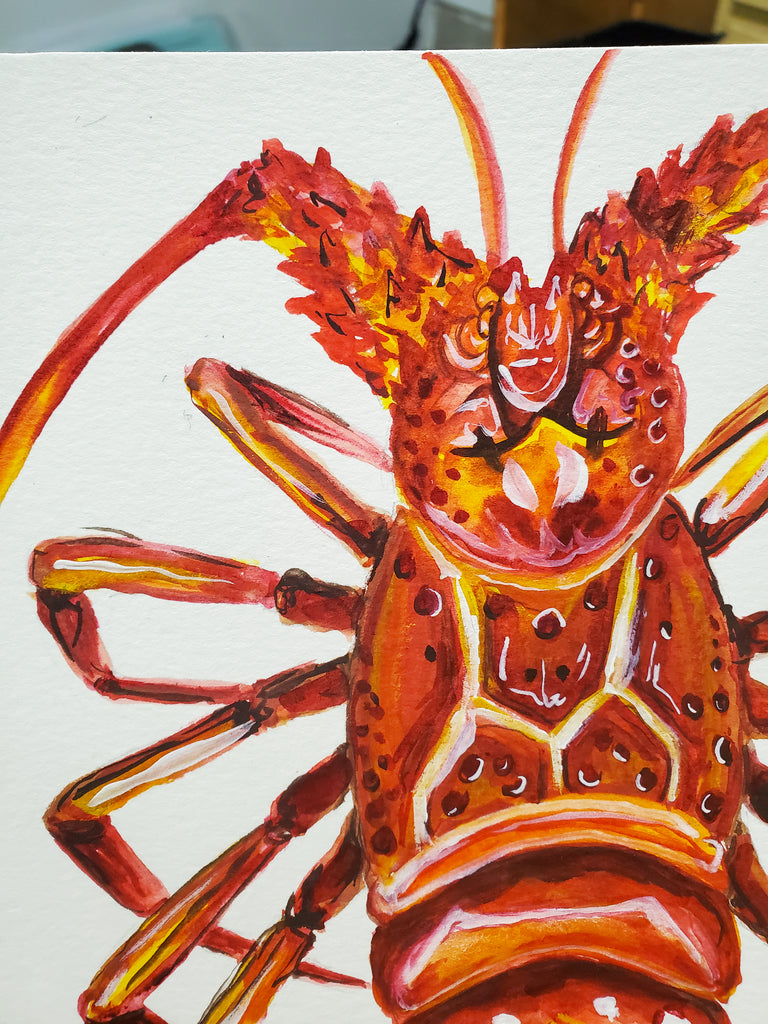The painting is a close-up of a lobster-like creature, portrayed against a predominantly white canvas. The artwork focuses on the upper three-fourths of the creature, with the right-hand side partially cut off. The lobster's body is a blend of deep reds, blacks, oranges, and yellows, with its antennae displaying hues of orange, yellow, and gold, accentuated with black. The intricate detailing on the creature showcases its scalloped tail and partial set of legs, with four fully visible on the left and partial ones on the right. Despite certain elements being ambiguous, such as circular marks on the body, the overall portrayal is vivid and dynamic, lending the impression that the creature is almost humorously posed, as if resting with one set of legs behind its back.